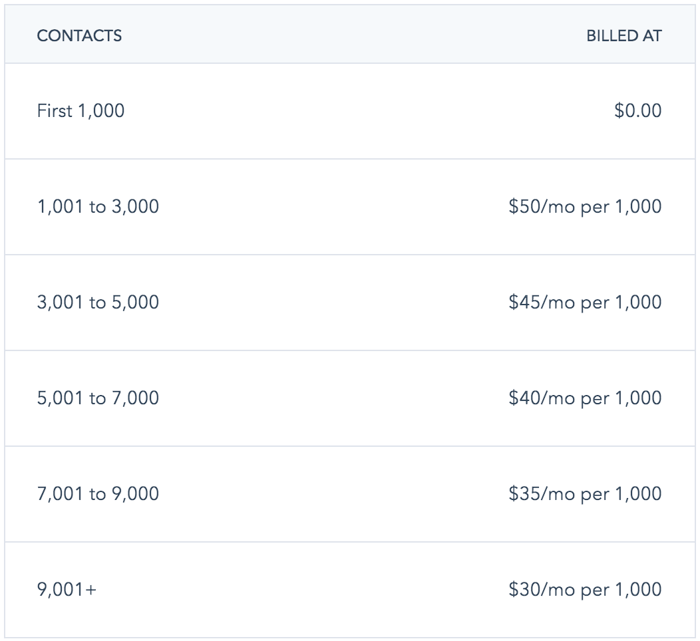The image features a table divided into two main categories: "Contacts" on the left and "Build At" on the right. The table is organized into rows, each row separated by very thin gray horizontal lines. The background at the top of the image is light gray, while the remainder is white.

### Contacts (Left):
- **1,000** contacts
- **1,001 to 3,000** contacts
- **3,001 to 5,000** contacts
- **5,001 to 7,000** contacts
- **7,001 to 9,000** contacts
- **9,001 plus** contacts

### Build At (Right):
- **$0.00**
- **$50 per month per 1,000** contacts
- **$45 per month per 1,000** contacts
- **$40 per month per 1,000** contacts
- **$35 per month per 1,000** contacts
- **$30 per month per 1,000** contacts

The table is designed with clarity and organization in mind, utilizing consistent, thin gray lines to demarcate each row, ensuring easy readability and distinction between each category and its associated data.